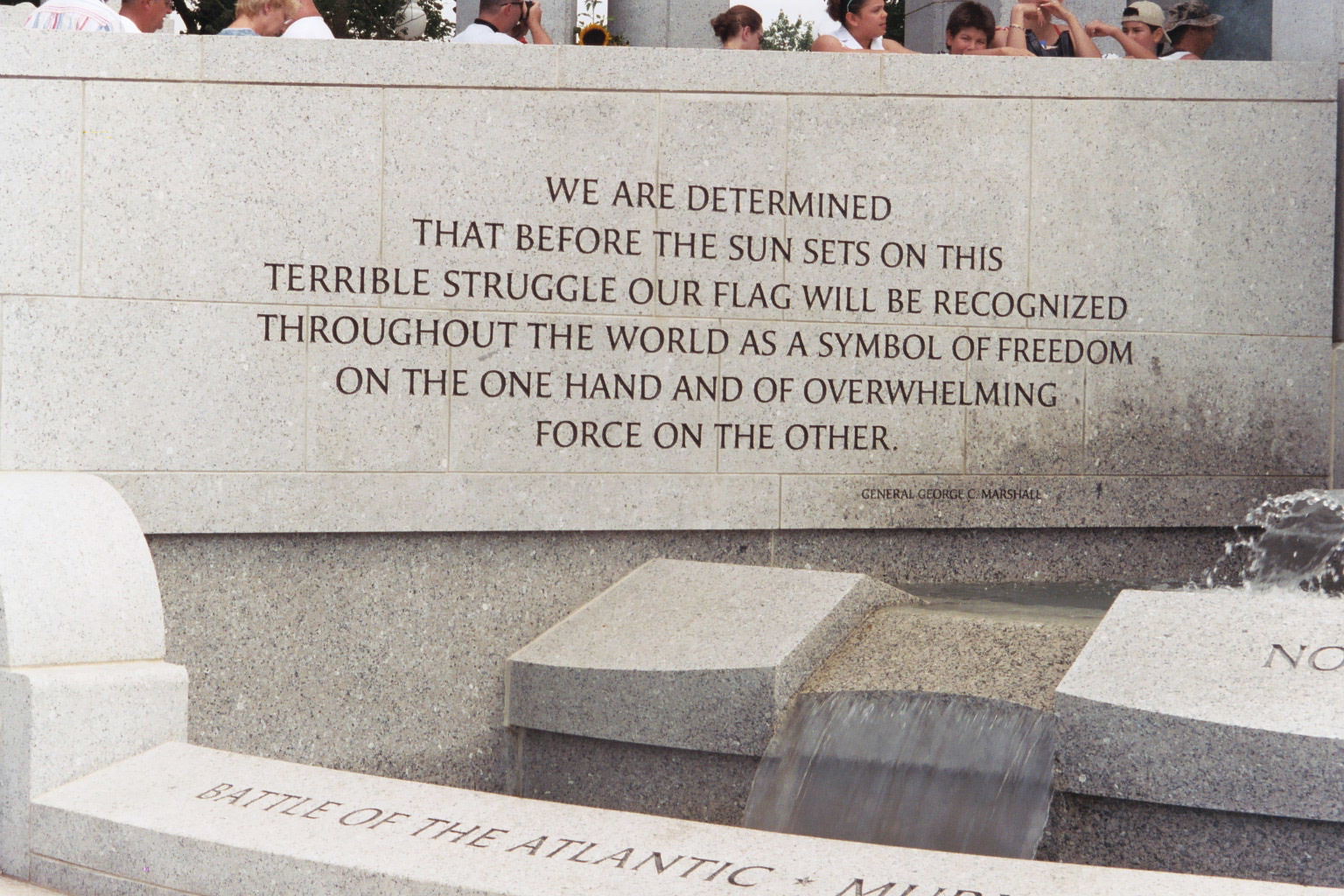The image depicts a large stone monument featuring a wall made of gray marble with black engravings. Dominating the center background of the scene, the wall bears an inscription that reads: "We are determined that before the sun sets on this terrible struggle, our flag will be recognized throughout the world as a symbol of freedom on the one hand and of overwhelming force on the other." attributed to General George C. Marshall. Below this prominent inscription, there is a smaller section of the monument with a marble slab that reads "Battle of the Atlantic." In front of the wall and slightly to the right, a small waterfall spills over a marble barrier. Above the wall, a group of people, possibly on a field trip, are visible taking pictures with cell phones, though they are only a small part of the overall image. Displayed across the bottom of the monument are several books or book-like structures contributing to the memorial's detailed and reverent design.